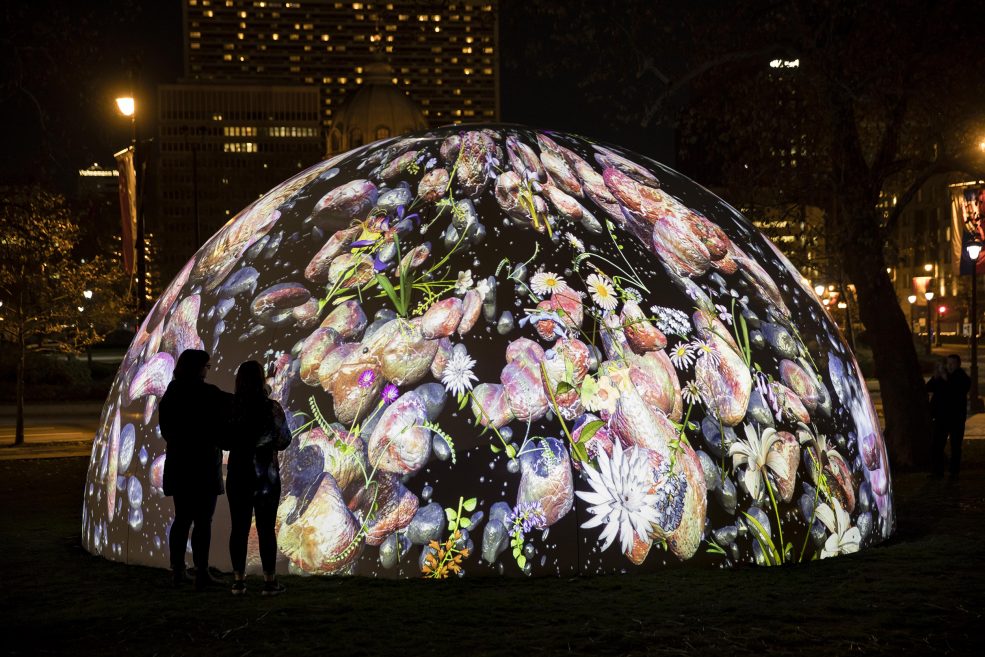This nighttime photograph captures a vibrant, illuminated half-dome artistic structure in a city setting. The dome, approximately 15 feet high and twice as wide, emerges from the ground, with only its top half visible. It stands out against the dark surroundings, glowing brightly with projections of white and pink flowers intermixed with green leaves. The dome's black background is peppered with tiny white dots, enhancing the striking floral imagery. Two silhouetted figures, likely women with long hair, are positioned to the left of the dome, adding a sense of scale and human presence. The dimly-lit scene includes a silhouetted tree in the foreground and, in the distance, the outlines of city buildings with glowing yellow windows. Scattered streetlights and additional buildings to the right suggest a downtown area, creating a captivating urban nocturnal landscape.